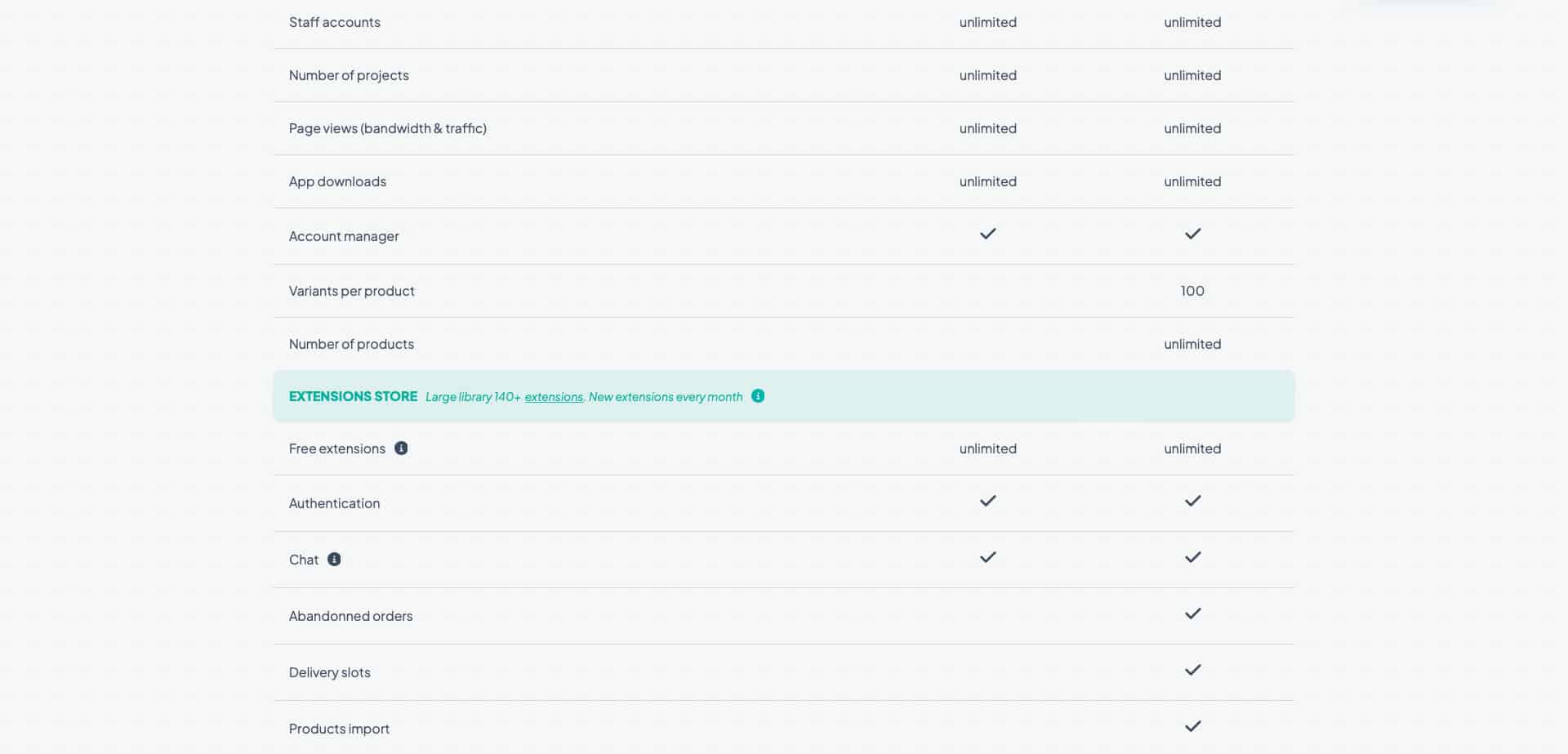This image is a detailed screenshot displaying the features of a business program, comparing a basic plan to a premium plan. The background is white, featuring black text, and in the middle section, there is a section titled "Extension Store" highlighted with a light blue background and teal text.

From the top, the image outlines various features included in both plans:

1. **Staff Accounts**: Unlimited
2. **Number of Projects**: Unlimited
3. **Page Views**: Unlimited
4. **Quotations**: Unlimited
5. **Bandwidth**: Unlimited
6. **Traffic**: Unlimited
7. **App Downloads**: Unlimited

Both plans also include an **Account Manager**. 

For the premium plan:
- **Variants per Product**: 100
- **Number of Products**: Unlimited

The image then highlights the "Extension Store" section.

Under this section, the following features are listed, common to both the basic and premium plans:
- **Free Extensions**: Includes a hover-over option to describe the extensions.
- **Authentication**
- **Chat**

After listing features common to both plans, the image concludes with premium-only features:
- **Abandoned Orders**
- **Delivery Slots**
- **Product Import**

This thorough comparison helps potential users clearly understand the benefits and capabilities of each plan, aiding in their decision-making process.